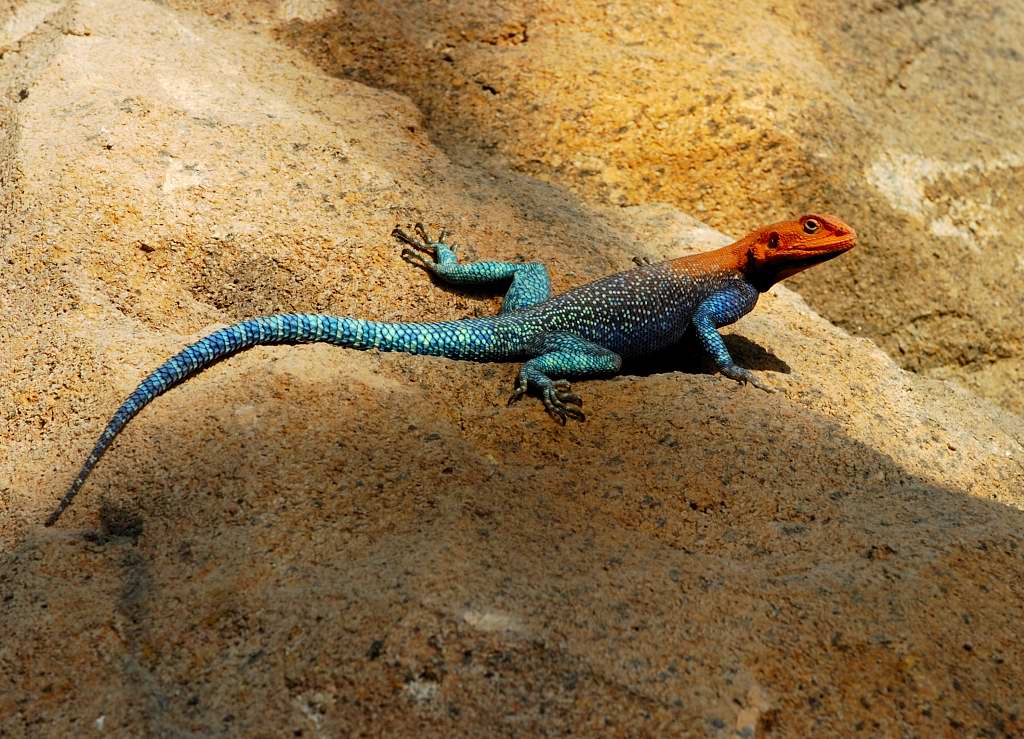This professionally captured, close-up photograph features a striking lizard prominently displayed in a horizontal orientation against a desert-like, rocky background. The setting includes a giant, yellow-gold rock peppered with patches of white and surrounded by sandy terrain, all shining brightly under the sun. The lizard, which seems to be possibly a chameleon due to its vivid coloration, occupies most of the image, making its impressive form and gradient colors highly noticeable. 

The lizard's body exhibits a remarkable color palette: its head and the top of its neck are a bright, fiery red, transitioning to a darker blackish-blue towards its midsection. The limbs and long tail are a vibrant turquoise, adorned with spots of bluish-green, creating an iridescent effect. The tail's hue deepens toward its end. The creature is captured in profile, its right eye focused on the camera, giving it a somewhat vigilant, poised look, as if ready to dash off at any moment. The sunlight accentuates its colors, adding to the high-definition clarity of this mesmerizing shot.